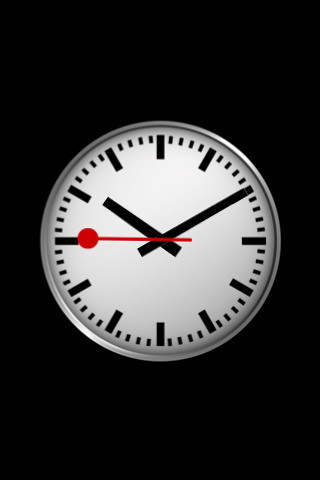This image depicts a clipart-style, computer-generated graphic of a circular analog clock on a solid black, vertically oriented rectangular background. The clock features a bright white face with a metallic silver outline. Instead of numbers, the clock face contains black rectangular bars at the positions where the numbers 1 through 12 would traditionally be. Thicker, shorter bars mark the minutes between these positions. The hour and minute hands are simple black straight lines, while the second hand is a thin red line ending in a small circular ball. The clock displays the time as 10:10, with the red second hand pointing to the 9.